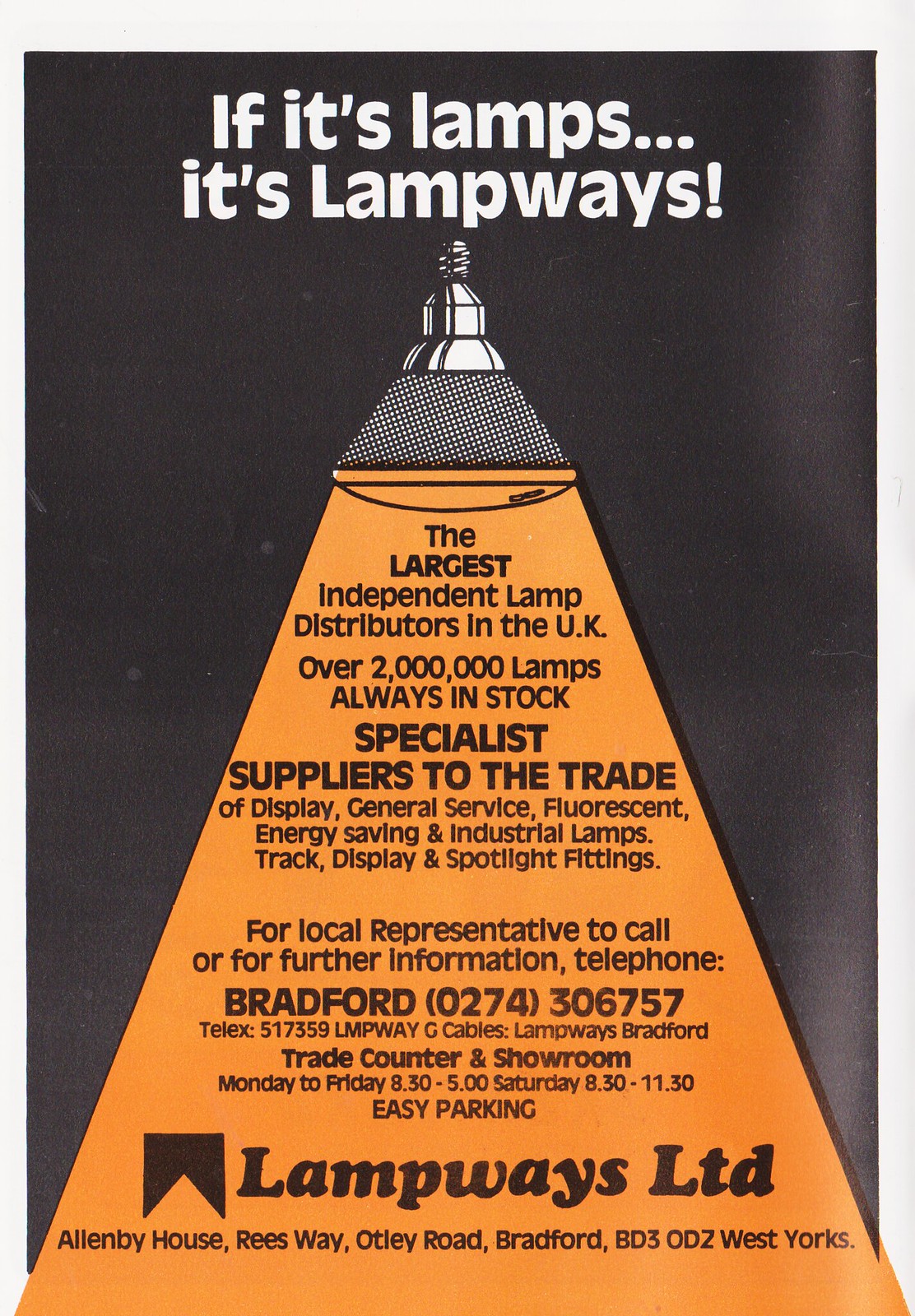The poster titled "If It Snaps, Dog, Dog, Dog, It's Lame Waste!" features a striking design with a black background and painted white text. Below the bold title, a large orange triangular section dominates the center, illuminating a message in black text. The focal point of the poster is an advertisement for Lame Waste Limited, showcasing them as the largest independent lamp distributor in the UK, with over 2 million lamps always in stock. They specialize in supplying display, general service, fluorescent, energy-saving, and industrial lamps, as well as track, display, and spotlight fittings. The ad emphasizes their professional service and extensive stock. At the bottom, contact details are provided, including a telephone number for Bradford (0274-306757) for further information or to reach a local representative. The company name, Lame Waste Limited, is mentioned again, underlining their brand identity.